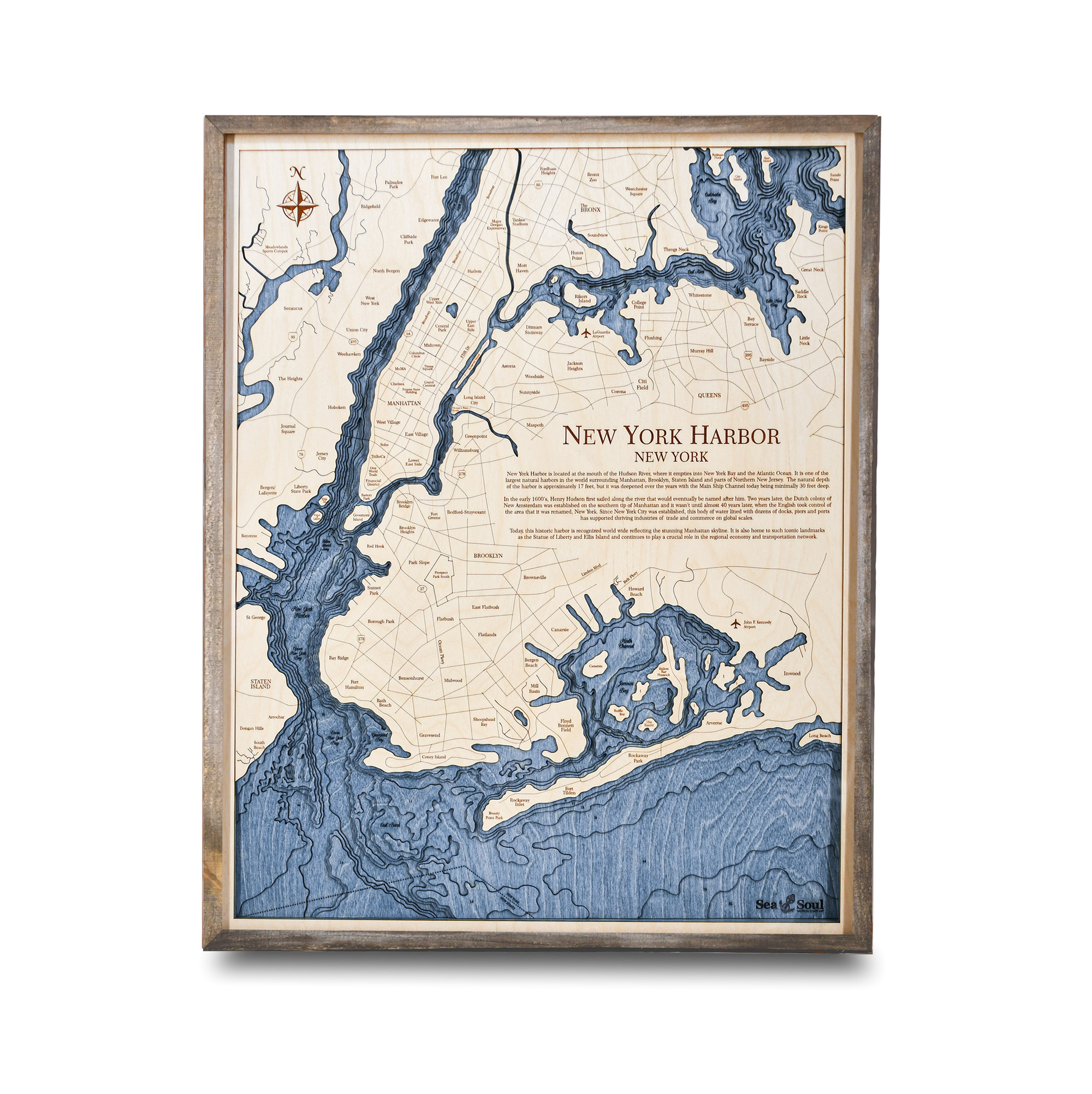This is a detailed map of New York Harbor in New York City, showcasing the land in a tan color and the waters in blue for clear differentiation. The map provides an intricate depiction of the harbor, including various inlets and other geographical features. Notably, it includes a section on the right-hand side containing a descriptive paragraph rather than a traditional key. Throughout the map, the names of what are likely boroughs are displayed, except in the area occupied by the descriptive paragraph. In the northwestern corner, a compass is present for orientation. The map also features lines, which might indicate water depths or possibly demarcate different areas of administrative control, potentially managed by state authorities.